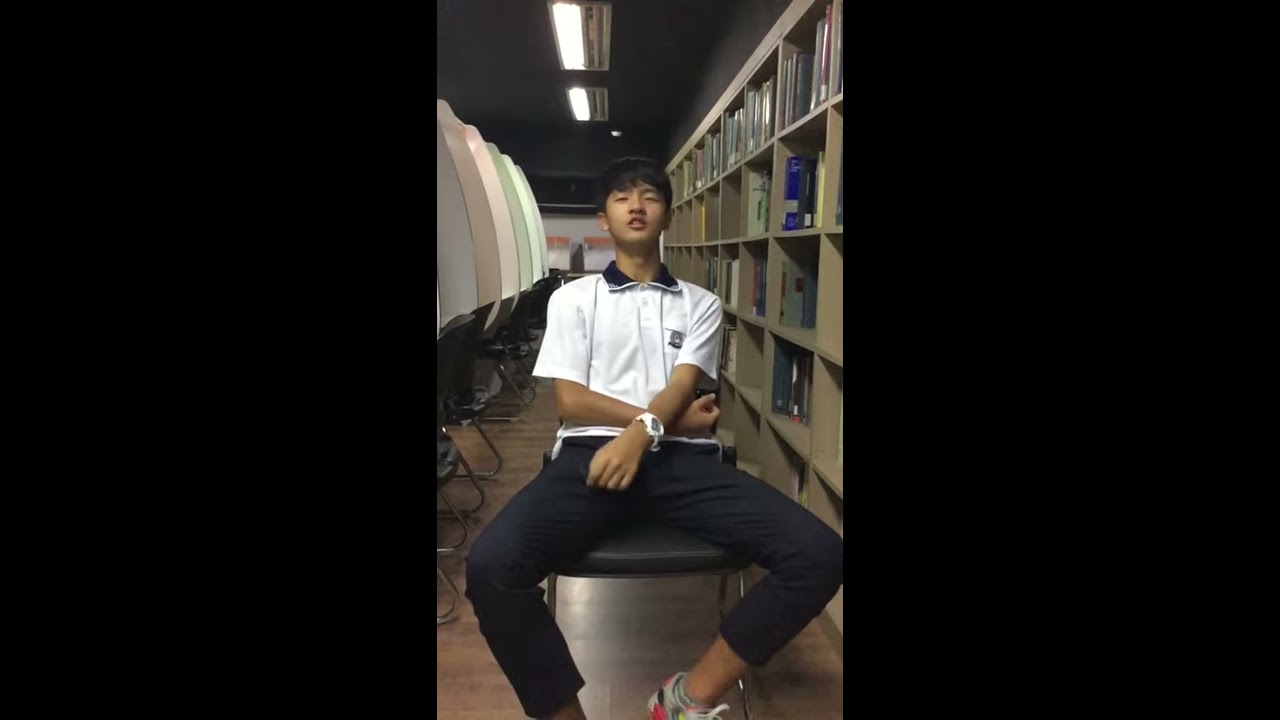A young Asian boy is sitting on a black chair in the center of a library-like room, facing and squinting at the camera. He has short dark hair and is dressed in a white polo shirt with a black collar and a logo on the left chest, along with blue or black pants, athletic shoes without socks, and a white watch on his left wrist. The setting features a wooden floor and a line of white study carrels with metal legs extending to the wall on his right. Behind him, there is a stretch of bookshelves reaching into the horizon and a distant white wall. Above, the ceiling is black with fluorescent lighting. The scene is devoid of any text, and the predominant colors include black, white, brown, red, gray, green, and blue, suggesting an indoor environment, possibly during the day, within an educational campus.